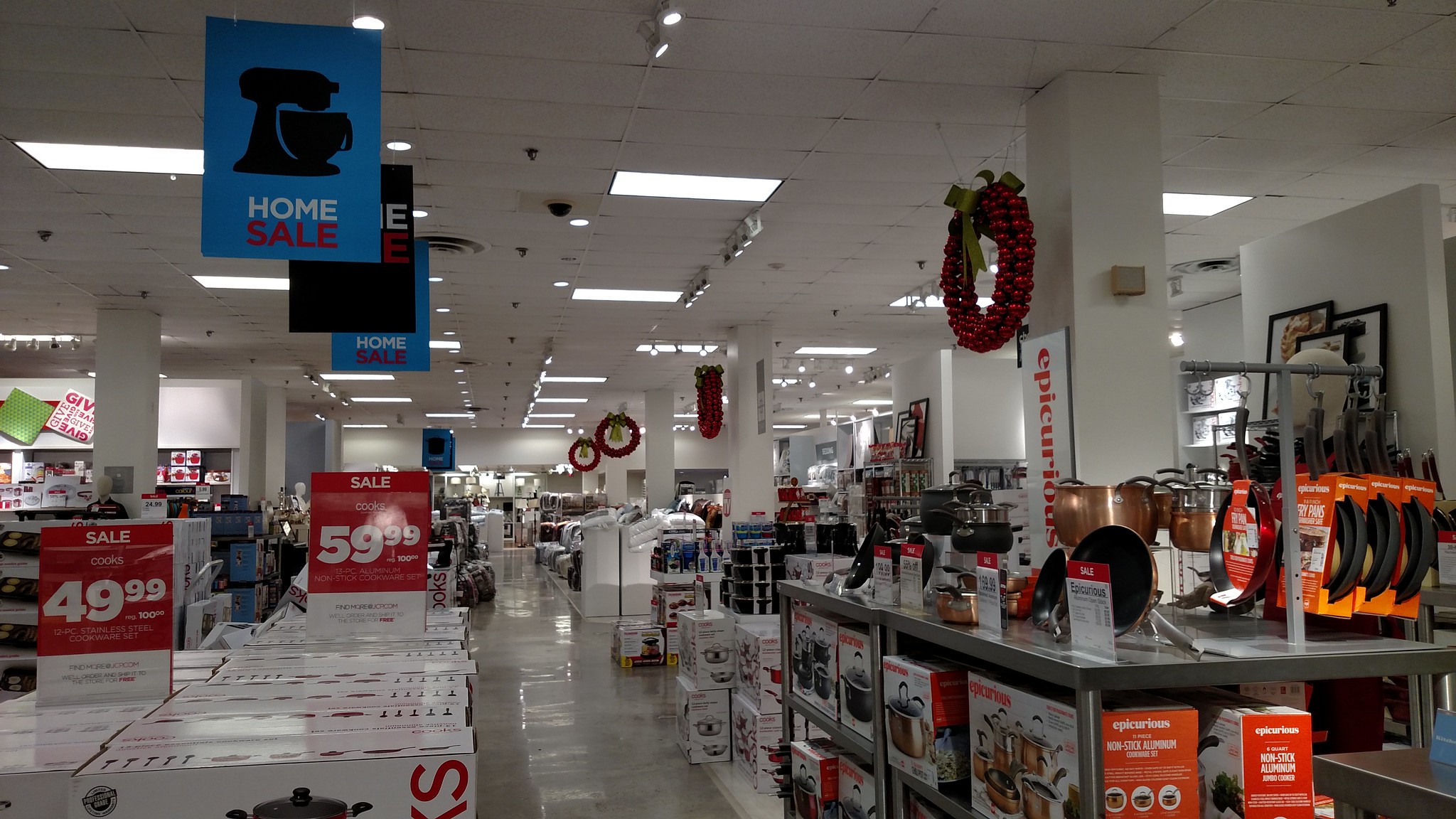The image appears to capture a section of a retail store's kitchen department, festively decorated for the Christmas season. Hanging from the ceiling are dark reddish wreath-like ornaments, each adorned with a decorative bow at the top. The shelving unit prominently displays an assortment of kitchenware: the top level features various pans, while the lower levels showcase pots with glass lids, each lid equipped with a handle.

In the upper left corner of the image, a blue sign with a vector graphic silhouette of a blender is visible. Below this graphic, bold white capital letters spell out "HOME," and underneath, the word "SALE" is prominently displayed in red capital letters. Partially obscured behind this is another mostly black sign with indistinguishable text. Further down, another blue sign reads "HOME SALE."

Among the items on display, several sales signs are noticeable, with one indicating a price of $49.99 and another marked at $59.99. The store's interior includes white pillars and a tiled ceiling, contributing to the clean and organized ambiance of the kitchen section.